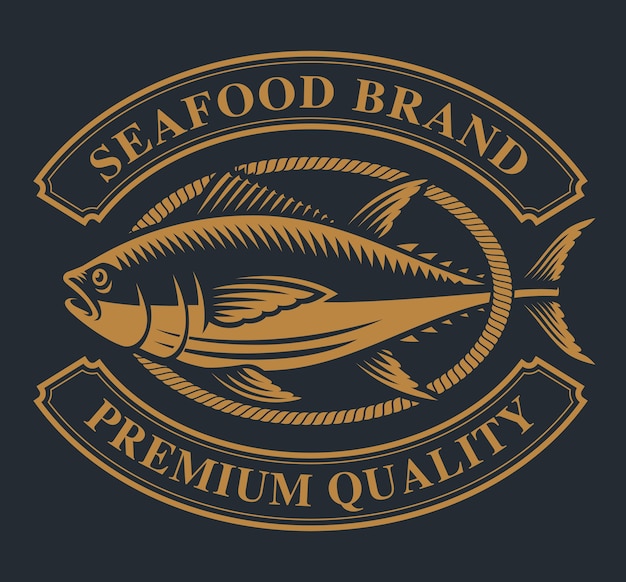The image features a meticulously designed logo set against a very dark gray, almost black background. The centerpiece of the logo is a fish rendered in a color that falls between burnt orange and brown, exhibiting a distinctive linoleum cut style with sharp, blocky angles. The fish, which resembles a bass with a modern, sleek, and sharp appearance, faces left and has partially overlapping colors due to the black background. Encircling the fish is a rope-like texture, adding a layer of intricacy to the design. Above the fish, a curved banner reads "Seafood Brand" and another curved banner below declares "Premium Quality." The precise and somewhat decorative details suggest that this could be a template or a portfolio project rather than the logo for an actual business.